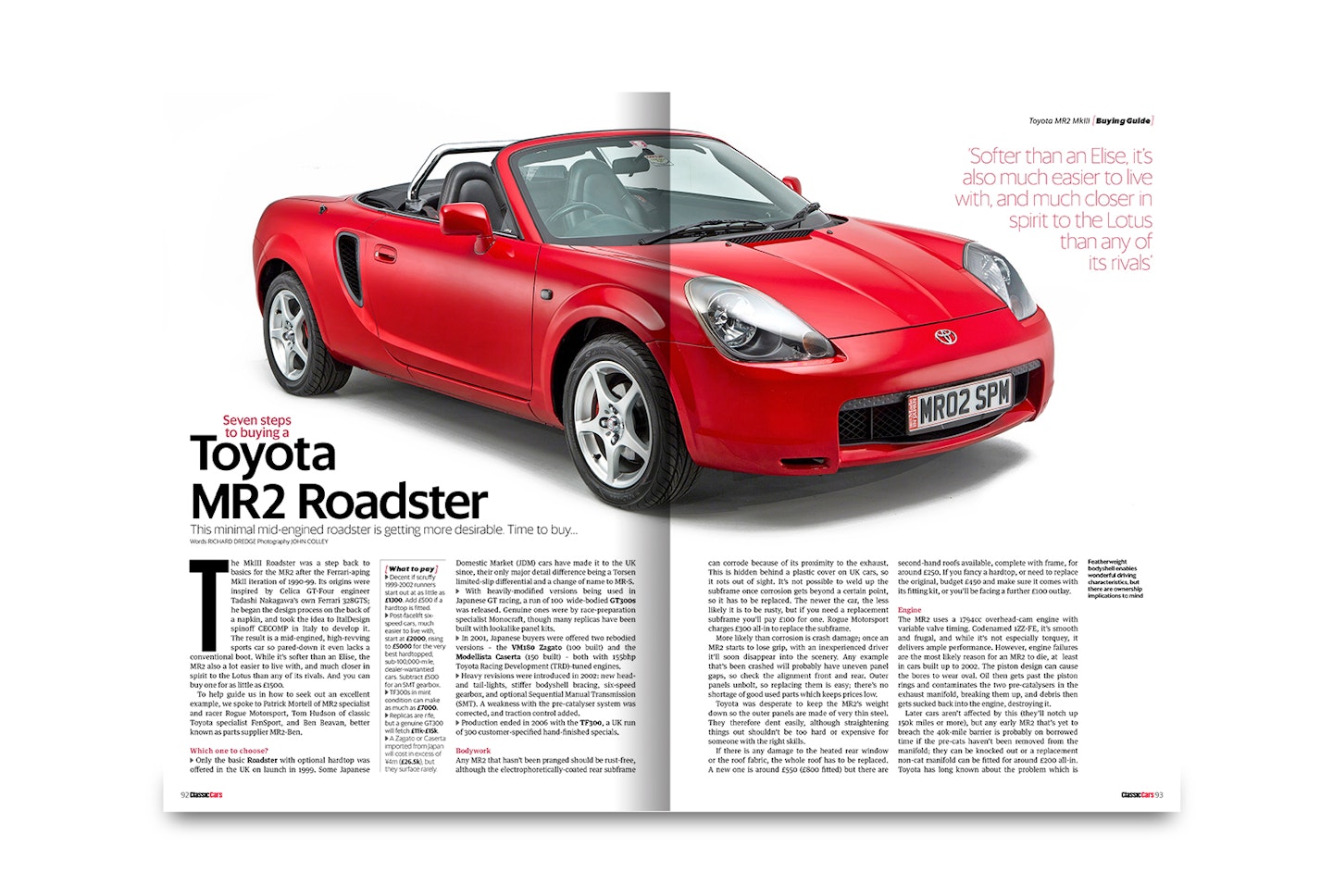This is a photo of a magazine centerfold featuring a detailed article about the Toyota MR2 Roadster. A striking deep cherry red, two-seat convertible sports car stretches majestically across the two pages. The top half of the spread is dominated by the image of the car, complete with large bug-like headlights, small silver five-spoke rims, and a noticeable U-shaped air intake on the side behind the door. The headline on the left page clearly states "Toyota MR2 Roadster," introducing the car enthusiastically. In the top right-hand corner, a quote in pink reads, "Softer than an Elise, it’s also much easier to live with and much closer in spirit to the Lotus than any of its rivals." Beneath the image, there are dense columns of text providing an in-depth review of the vehicle, though too small to read from the photo alone. Additionally, the lower left corner highlights "Seven steps to buying a Toyota MR2 Roadster," prompting readers to delve deeper into their exploration of this exciting model. The entire layout exudes speed and elegance, captivating any car aficionado’s attention.